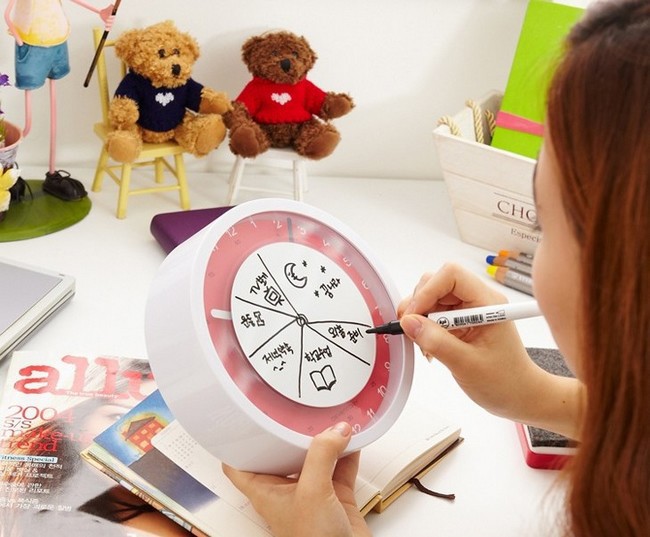A detailed caption for the image could be:

"A young woman with reddish-brown hair, appearing to be of Asian descent, sits at a pristine white desk, engaged in the creative process. Her pale skin contrasts with the white surroundings, including the wall behind her. She is meticulously drawing on a white piece of paper that covers the surface of an analog clock with a red face. The clock features a white circle divided into sections, adorned with writing in an Asian language, and she is adding details with a marker.

To her right, the clutter on the desk includes a stack of magazines, a purple binder, a black and white notebook, and a collection of thick, silver pencils with varied colored tips. A small white container houses a green book. On the left side of the desk, two teddy bears are seated on small stools; one bear wears a black shirt and the other a red shirt, both shirts displaying white hearts. Beside the teddy bears is a figure of a person, further adding to the eclectic assortment of items. The scene captures a moment of focused creativity amidst a setting filled with personal and colorful objects."